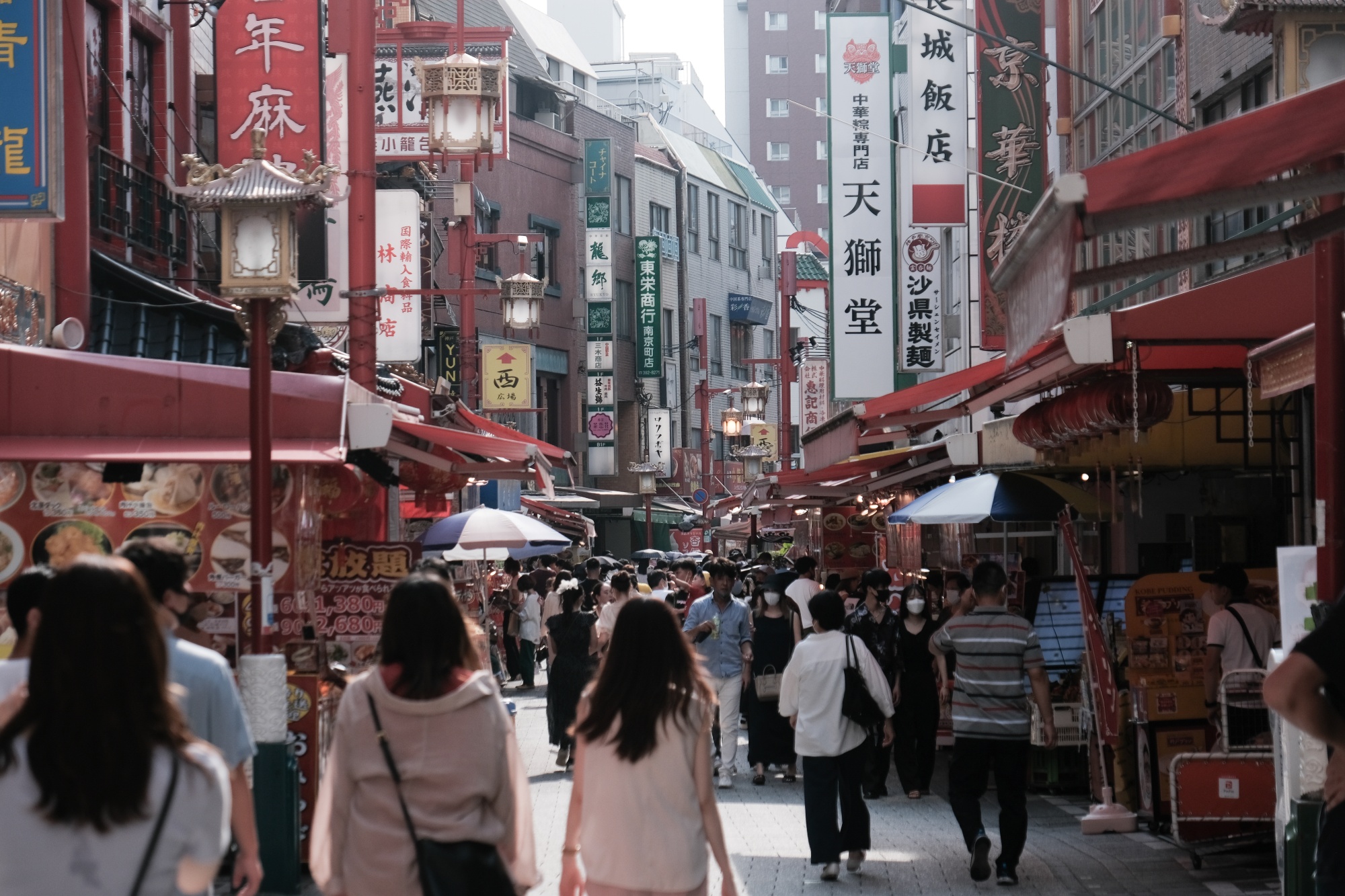The image depicts a bustling city street in what appears to be an East Asian country, possibly Japan, Korea, or China. The scene is packed with people navigating a narrow alleyway flanked by tall, tightly packed buildings adorned with numerous signs featuring Asian symbols, with no English in sight. Brightly colored red awnings extend from the sides of the shops, beneath which are various food stalls and restaurants. On the left side, menus with pictures and prices are visible, suggesting the presence of eateries. There are also outdoor seating areas with small umbrellas. The crowd, a mix of individuals carrying bags and purses, moves both towards and away from the camera, contributing to the vibrant atmosphere. In the foreground, there’s a notable design feature that resembles a lantern but might serve a decorative purpose. The cityscape in the background showcases tall buildings with many windows, reinforcing the image of a busy urban environment.